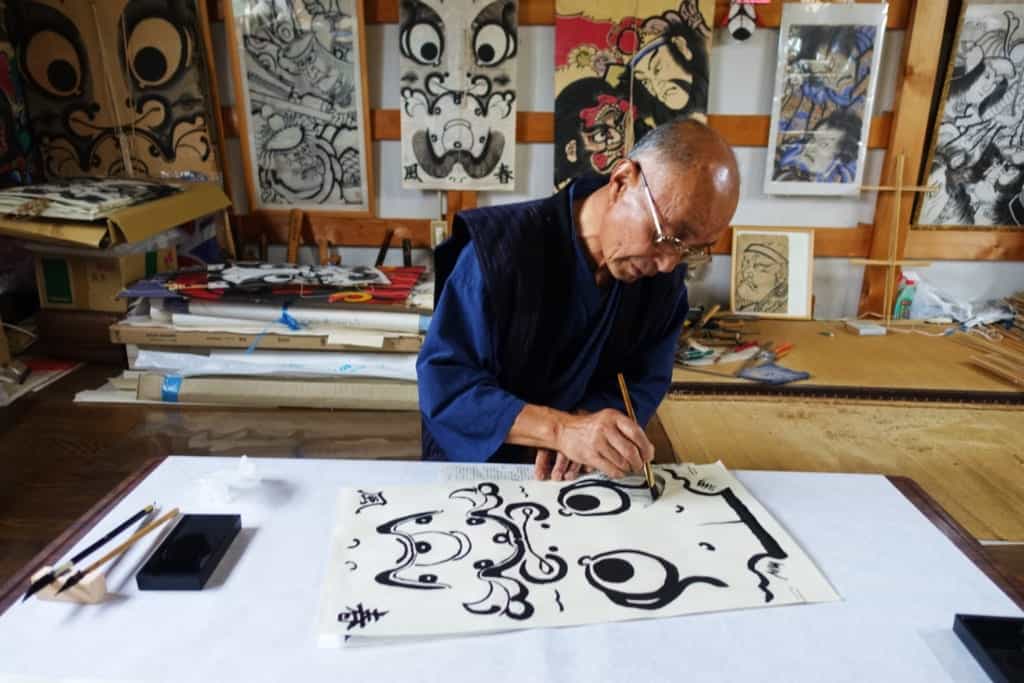In this detailed indoor photograph, an artist stands in his cluttered studio, intensely focused on his work. He is attired in a blue shirt with a darker blue cotton vest over it. The artist, who appears to be of Oriental descent, is nearly bald and wears glasses. He holds a paintbrush in his right hand, steadily painting black, expressive lines on a white canvas laid out on the table before him. The artwork in progress features two large eyes with intricate details forming around them, possibly an eyebrow being worked on. The table in front of him is covered in a white material and holds an eraser, two pens, and a small box for organizing his brushes.

Behind the artist, the floor space is occupied by a tall stack of canvases yet to be used. The back wall of the studio is adorned with a multitude of prints and pictures, showcasing a variety of his completed works. Some of these artworks resemble the one he is currently painting, featuring similar large eyes and intricate facial designs, while others vary in style and color, some in vivid hues and others in stark black and white. A brown counter at the back holds additional materials, hinting at a well-used and creative workspace. The overall scene captures the artist deeply immersed in his craft amidst a backdrop of his diverse and expressive creations.